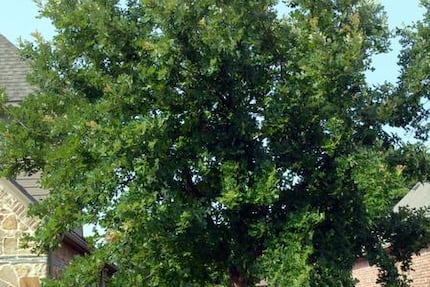This photograph captures a close-up view of the lush, green leaves of a tree with the backdrop of a lightly clouded blue sky peeking through. Situated in what appears to be a residential backyard, the tree is framed by partially visible houses on either side. To the left, a segment of a house is discernible, showcasing its tan stone walling and grey roof. On the right, another structure is faintly seen, also featuring brown-colored walls. The vivid colors of the image include shades of green from the dense foliage, patches of sky blue, and various earth tones from the buildings. The scene, likely photographed in spring or summer, conveys a tranquil, vibrant outdoor setting, although the exact type of tree remains unidentified.